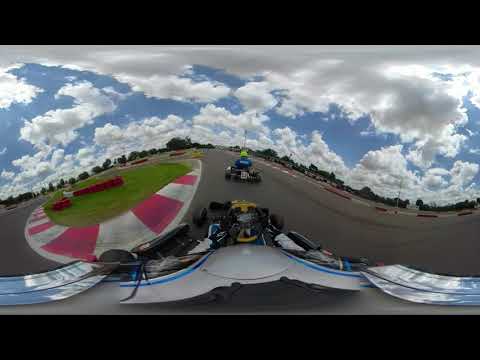In this detailed outdoor image, we see a segment of a go-kart racing track, captured from a first-person perspective as if the viewer is in one of the go-karts. The asphalt track stretches from the bottom center of the image and appears to curve off to the left, marked with red and white cement barriers that indicate turns. This dynamic shot, possibly taken with a GoPro or similar camera, gives the scene a distinctively warped, circular feel. 

At the bottom of the image, we can see parts of the front of the go-kart that holds the camera. This go-kart has a whitish body with blue striping and some yellow markings. The track itself is gray and black, with warning stripes on either side and patches of green grassy areas adjacent to it. The scene is bright, suggesting it was taken during the middle of the day with the blue sky above dotted with numerous clouds.

Additional drivers in other go-karts are visible ahead, with one driver in the center wearing a green hat and a blue shirt. Despite the apparent motion and excitement, there is no text in the image. Color accents include red and white on the track’s markings, and we notice some subtle pink on the track, possibly from lighting or lens effects. The image's overall effect is enhanced by virtual reality or camera-induced warping, making the track and surroundings visually engaging and dynamic.